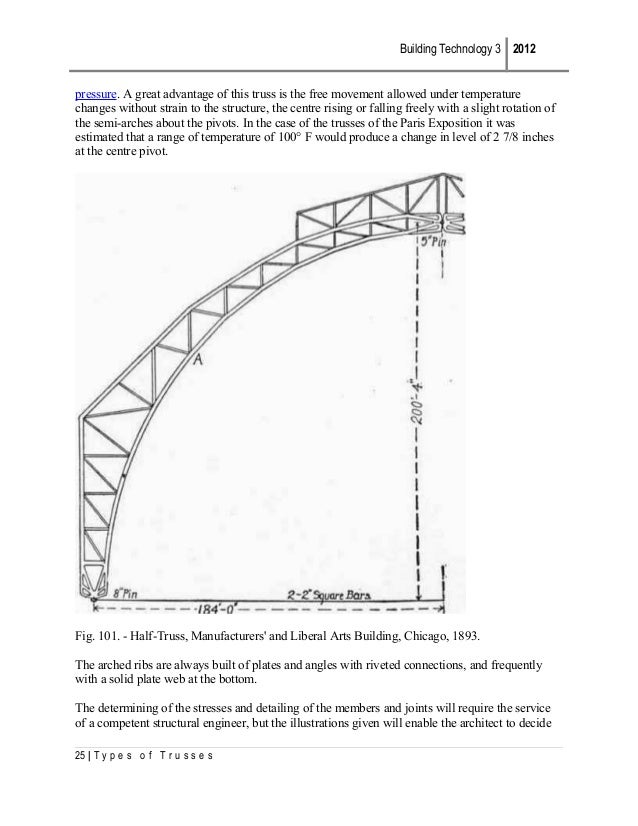The image features a blueprint-style diagram of a building truss, likely from a textbook or manual dated 2012, titled "Building Technology 3." The page is labeled as Figure 101 and is found on page 25 under the section "Types of Trusses." The diagram depicts the left half of a truss, highlighting its design and measurements. Text at the top right discusses the advantages of this truss type, particularly its ability to accommodate temperature-induced expansions and contractions without straining the structure. This is exemplified by a historical reference to the trusses used in the Paris Exposition, where temperature variations of 100 degrees Fahrenheit could result in a 2⅞ inch shift at the center pivot. Additional information at the bottom of the page includes the structural details, such as the use of plates and angles with riveted connections and a solid plate web at the arch ribs' base. The description emphasizes that the stress determination and detailed joint design require a competent structural engineer, although the illustrations support the architect's understanding. The truss is also associated with the Manufacturers and Liberal Arts Building in Chicago, 1893, possibly indicating its historical significance.